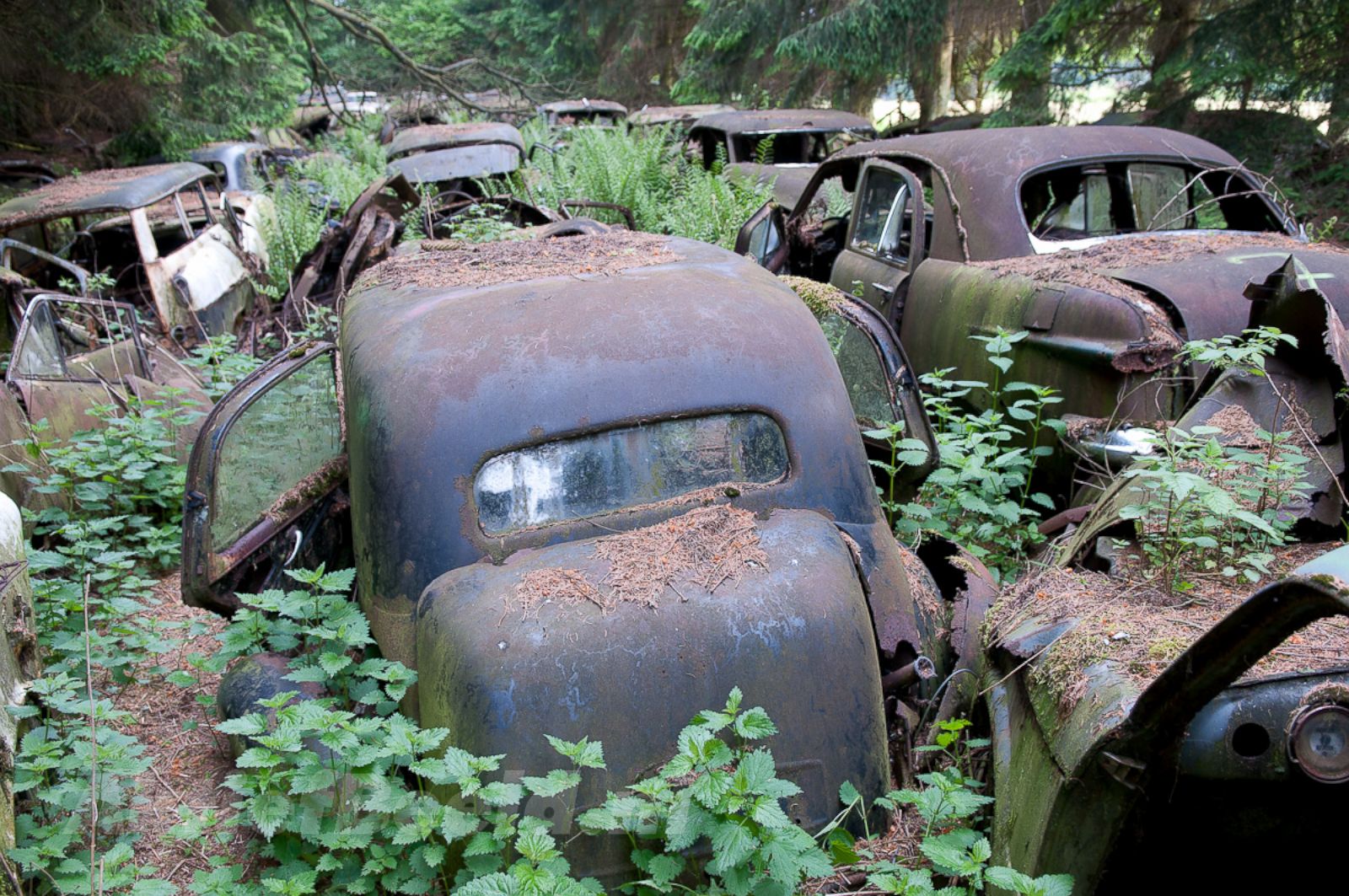In this photograph, a desolate junkyard teems with a multitude of antique cars, dating back to the 1920s through 1940s. These abandoned vehicles, numbering at least 15 to 20, stand in rows, ensconced within a dense, forested area. Rust blankets each car, rendering them a uniform orange-brown hue, while dirt accumulates on their surfaces. Many of the cars feature broken windows, open doors, and popped trunks, revealing interiors in disarray. Some gauges are missing, leaving empty holes on the dashboards. Verdant greenery, comprising weeds and grass, has grown unchecked, even reaching up to the roofs of some cars. The scene is a mosaic of decay and reclamation by nature, with sunlight barely filtering through the thick canopy of trees surrounding this secluded, forgotten site.